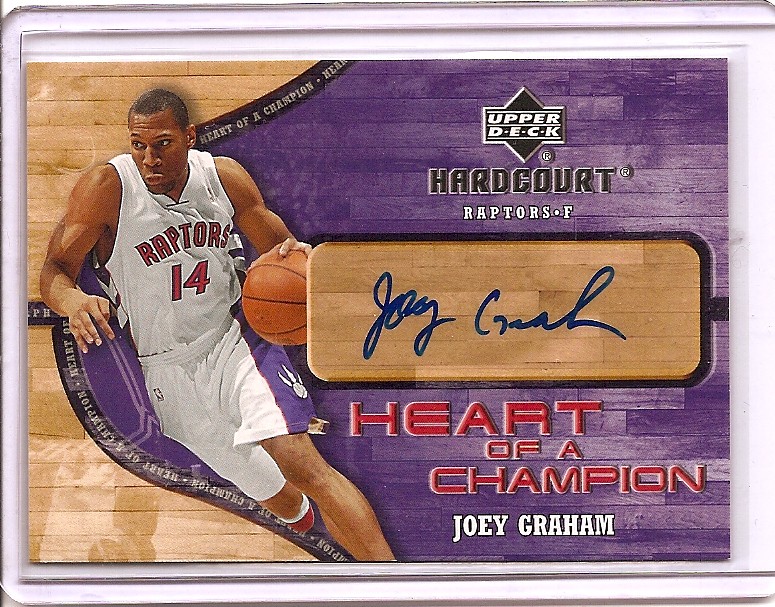This color photograph showcases a meticulously detailed sports trading card featuring basketball player Joey Graham. The card, branded by Upper Deck and labeled "Hard Court," prominently displays the Raptors' forward. Joey Graham, an African-American athlete, is depicted in action on the left side of the card, dribbling intensely while wearing a white Raptors jersey with red number 14 and long shorts that feature a purple stripe and the Raptors logo. The card's design juxtaposes a rich purple basketball court background with natural hardwood floor elements in the corners, enhancing its visual appeal. 

The center of the card features Joey Graham's autograph, set against a background reminiscent of a basketball court floor, giving it an embossed, tactile quality. Below the signature, in bold red text, reads the motivational phrase "Heart of a Champion," followed by Joey Graham's name in print. The card is encased in a clear protective sleeve, highlighting its value and preserving its condition. Every element, from the finely detailed illustration of the player to the embossed text elements, contributes to the card's premium feel, making it a prized collectible for any basketball enthusiast.